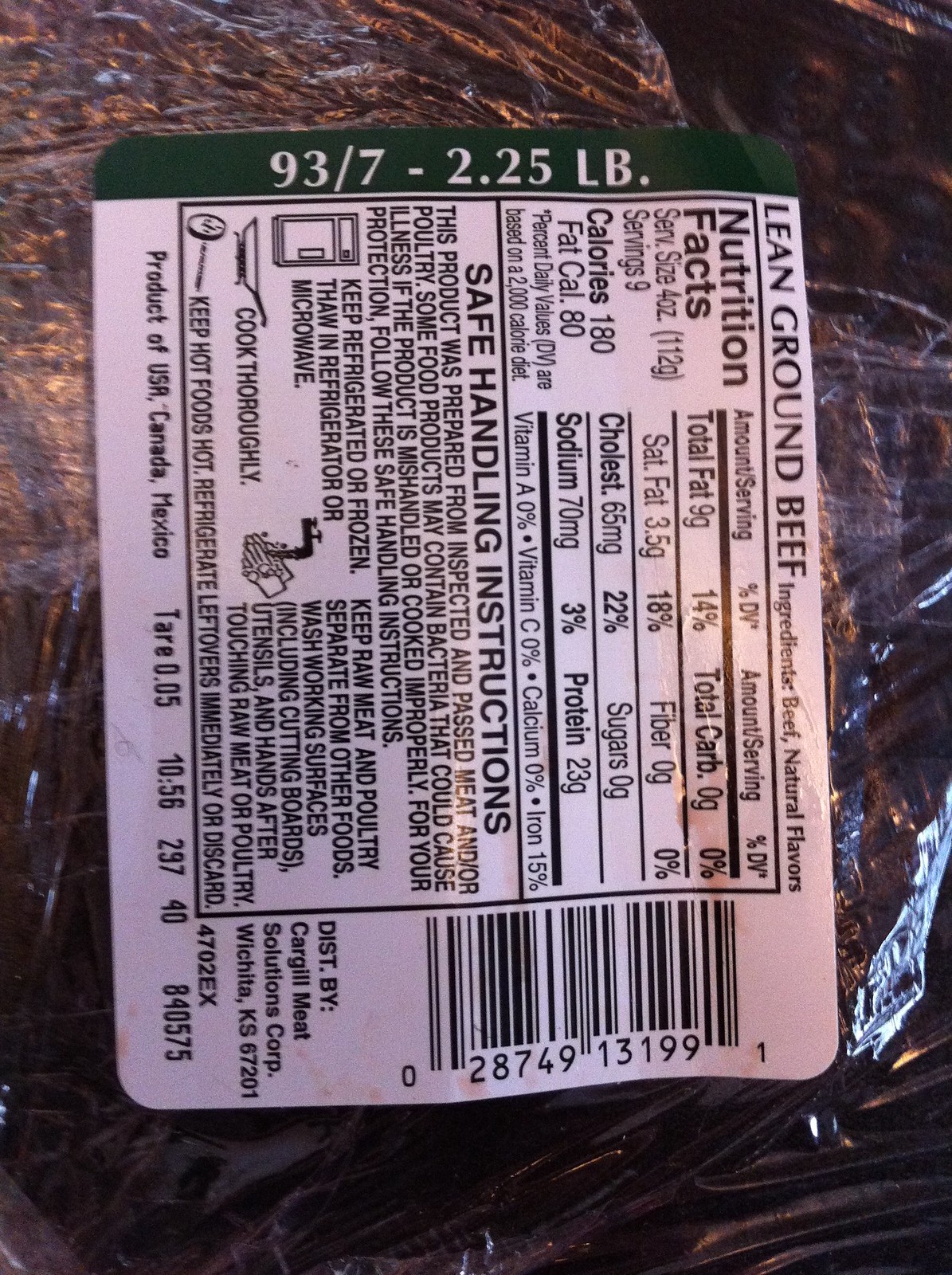This image depicts the back label of a package of lean ground beef, placed vertically so that reading it requires tilting your head sideways. The label, affixed to a Saran Wrap-type film covering the beef, prominently features "Lean Ground Beef" at the top. Just below, it lists the ingredients as beef and natural flavors, noting that the beef is 93% lean and 7% fat. The label includes a nutrition facts box followed by a section dedicated to safe handling instructions. On the bottom left, it states "Product of USA, Canada, Mexico," while the weight information, displayed in large white letters, appears both at the bottom right and in a black box along the side of the label. Additionally, a clearly visible barcode is located at the top right corner of the package.